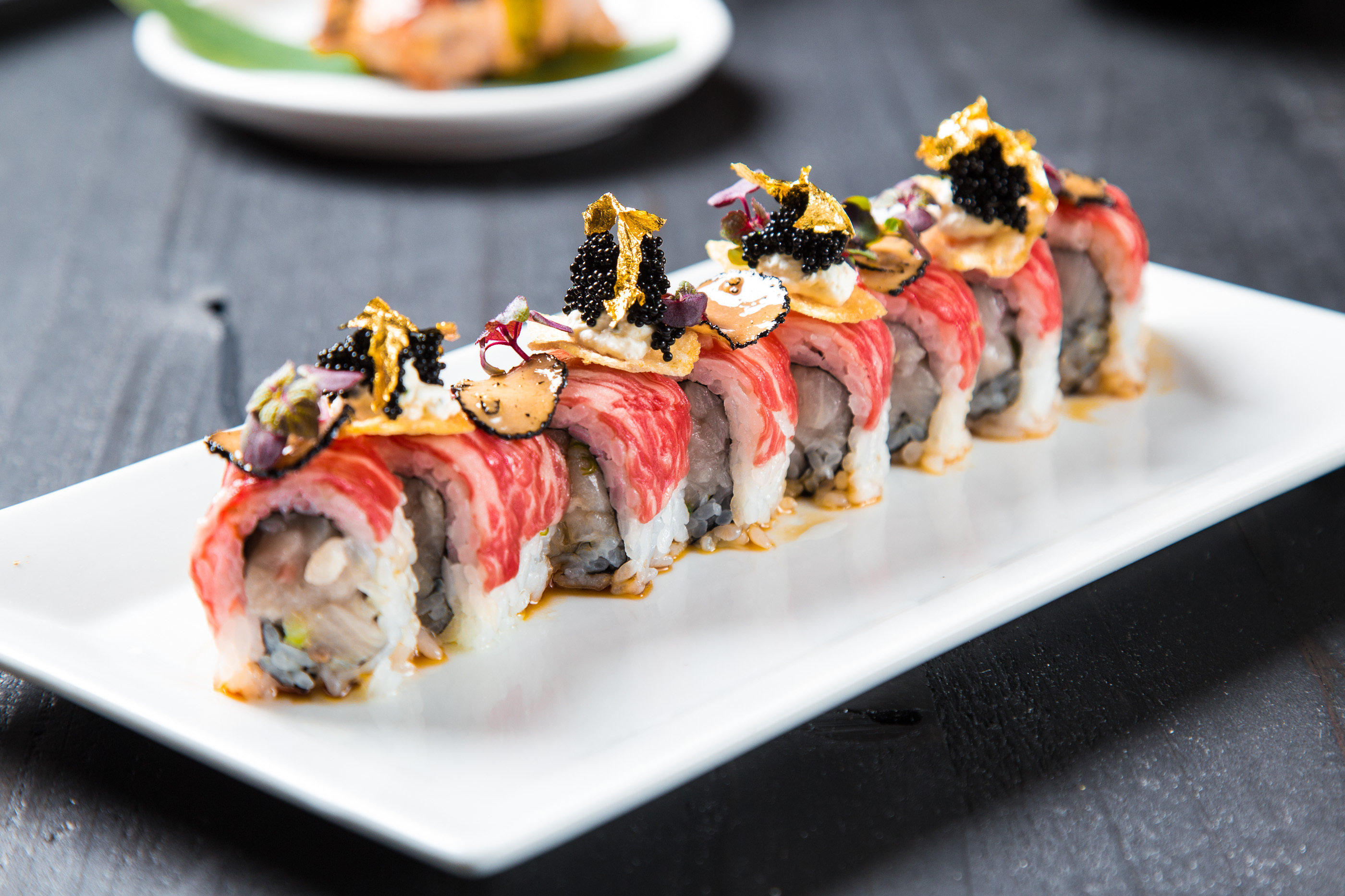The image features an upscale dining setting with a finely presented serving of sushi, placed in the center on a small, rectangular white plate, typical of those found in high-end seafood restaurants. The sushi is expertly sliced and showcases a vibrant red exterior with intricate fillings that include small black seeds or sesame seeds. Nestled within the sushi pieces are delicate black caviar pearls. Adorning the top of the sushi, there appears to be fragments of yellow, chip-like garnishes, possibly gold leaf, adding an extra touch of luxury. Surrounding this main dish is a spread of additional culinary creations on similar white plates, all set against a wooden table with a grayish-black hue. The colors in the sushi dish are striking, with hues of pink, red, yellow, and black, contrasting against the blurred greens and oranges of the background plates.